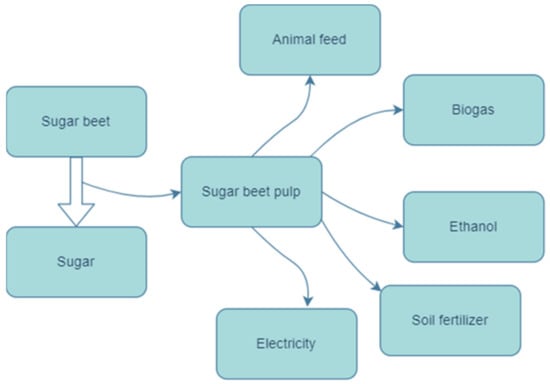The image is a detailed flowchart illustrating the various products derived from a sugar beet. The flowchart consists of eight horizontally rectangular pieces bordered in dark blue, with dark blue text against a light blue background. Starting at the top left, the first rectangle is labeled "sugar beet" and has a downward arrow pointing to the next rectangle, labeled "sugar." Additionally, there's a horizontal arrow from "sugar beet" pointing right to another rectangle labeled "sugar beet pulp." From "sugar beet pulp," five separate arrows radiate outward to five other rectangles, each designating a different product: "animal feed," "biogas," "ethanol," "soil fertilizer," and "electricity." This visually demonstrates how sugar beets can be processed into sugar and further utilized to produce multiple other forms of energy and products.